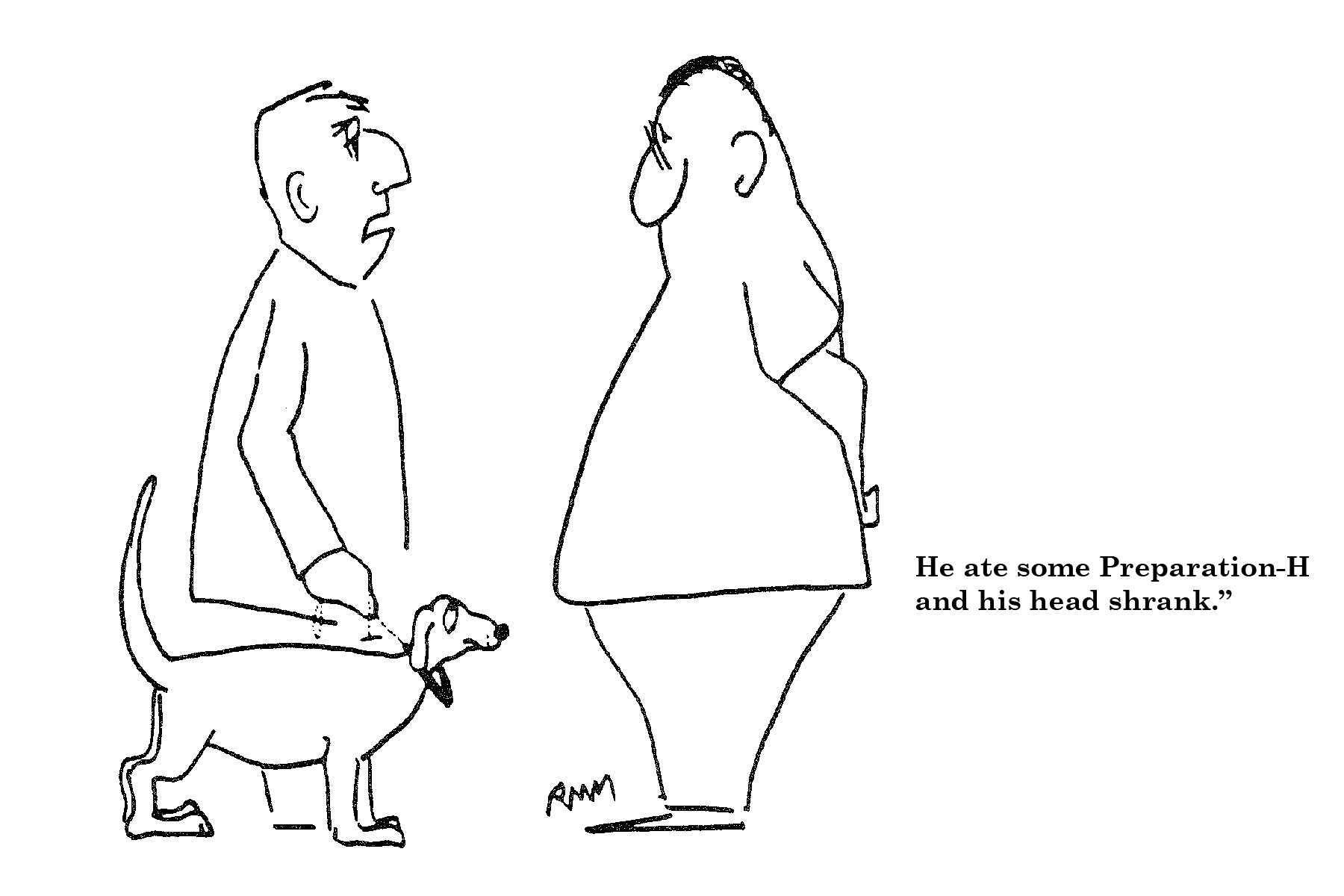In this cartoon sketch on a white background, two men are depicted in profile with simple black outlines. The man on the left appears older, characterized by a large, hooked nose, open mouth, and sparse hair combed forward. He is wearing a long-sleeved shirt and is holding a leash attached to his dog. The dog has a small head with a black-tipped nose, eyes looking upward, and a raised tail. The man on the right is obese with a droopy nose, short hair, and possibly glasses. His arms are clasped behind his back. The caption beside him reads, "He ate some Preparation H, and his head shrank." The comic is signed "R.M.M."